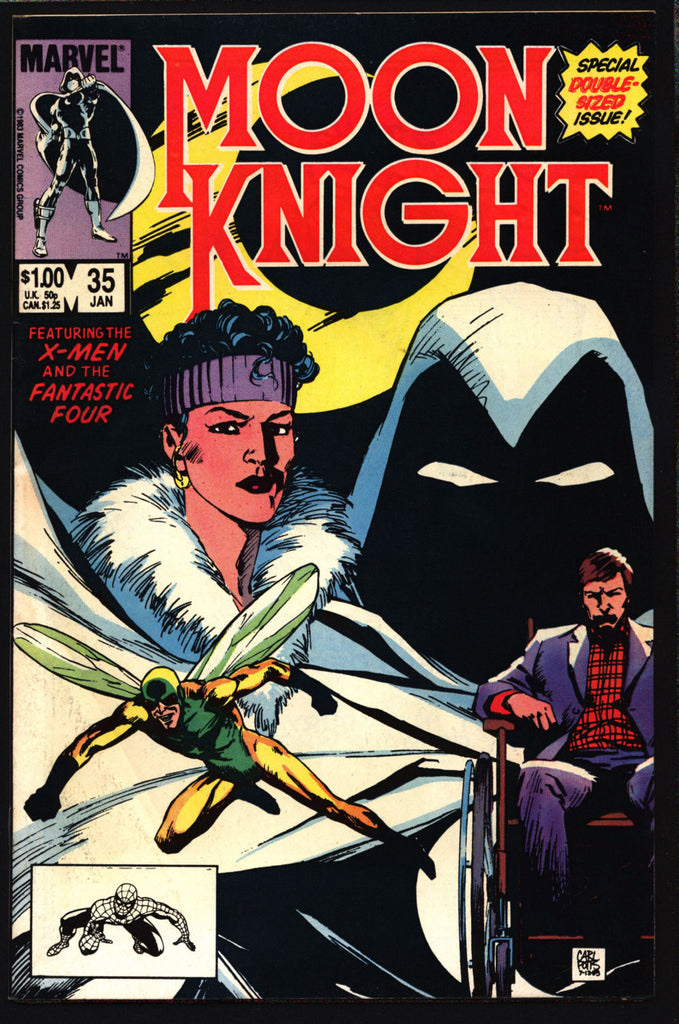The front cover of the 1983 Marvel Comics issue titled "Moon Knight" prominently features the title in red letters at the top, set against a backdrop of a crescent moon. The central figure in the artwork is Moon Knight himself, cloaked in white with only his eyes visible beneath a hood that points forward. Superimposed in front of Moon Knight are three distinct characters: a superhero resembling a wasp clad in yellow and blue; a man in a wheelchair positioned to the right; and a young woman with a headband and fur coat gazing at the viewer on the left. Additionally, on the lower left corner of the cover, there's a black and white drawing of Spider-Man.

Furthermore, the upper left corner of the cover announces the inclusion of the X-Men and the Fantastic Four, and a small image of Moon Knight is also present in this section. A banner on the upper right highlights that this is a special double-sized issue, priced at one dollar. The entire cover is illustrated in color, encapsulating a vivid and dynamic scene characteristic of Marvel's 1983 era.